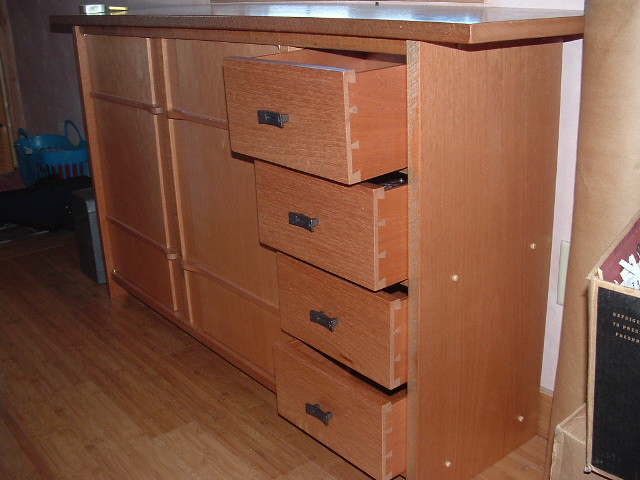This image showcases a long dresser situated on a light brown, laminated wood floor. The dresser, illuminated by a shimmering brown tabletop, features four columns of drawers, with the column closest to the viewer having its four drawers pulled out slightly. These drawers, interconnected with dovetail joinery and equipped with black metal handles, reveal meticulous craftsmanship. To the right of the dresser, a prominent black box with a brown trim is visible, positioned beside a roll of brown paper. At the dresser's front corner, a dark square object is noticeable. In the background, against the wall, a small plastic tote with two plastic handles and open slots further complements the setting.